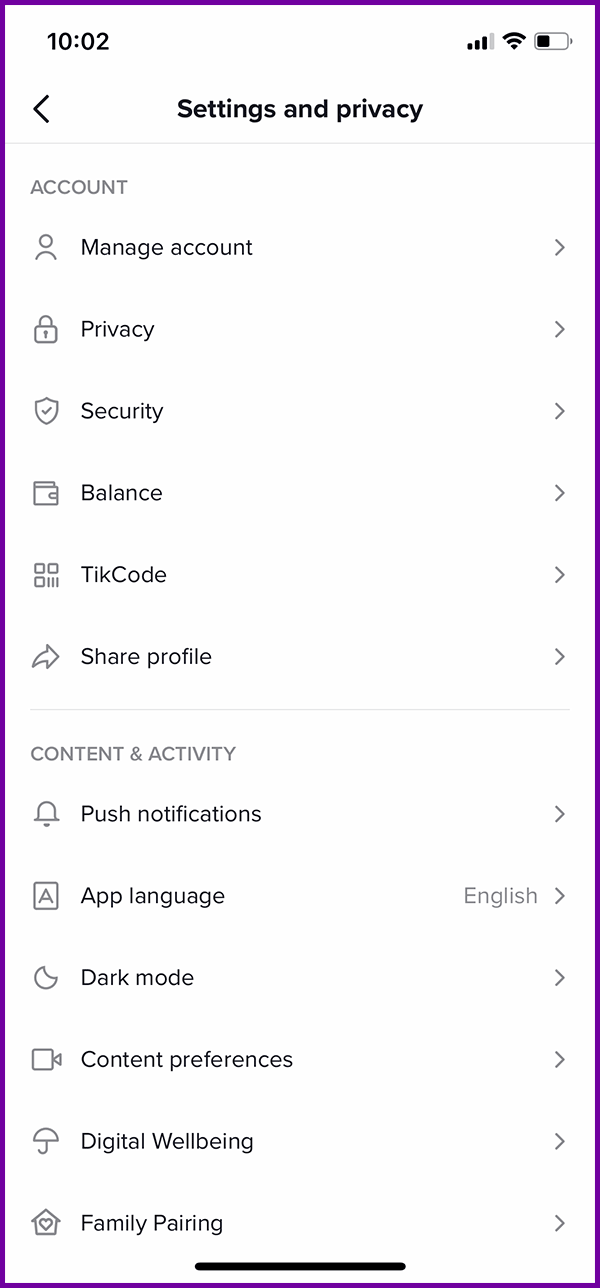A screenshot displays a smartphone interface at 10:02, featuring a full signal and approximately 25% battery remaining. The screen showcases a settings menu with the header "Settings and Privacy." Underneath, there are options listed as "Account," "Manage Account," "Privacy," "Security," "Balance," "QR Code," and "Share Profile," each accompanied by an arrow pointing to the right, indicating they are clickable.

Further down, the categories "Content and Activity" and "Push Notifications" are presented. The "App Language" option indicates "English" on the right side. Additional settings include "Dark Mode," "Content Preferences," "Digital Wellbeing," and "Family Pairing." The bottom of the menu is demarcated by a bold black line beneath "Family Pairing," suggesting it marks the end of the options.

The entire menu is enclosed within a light purple outlined box, with all settings listed within a black background.